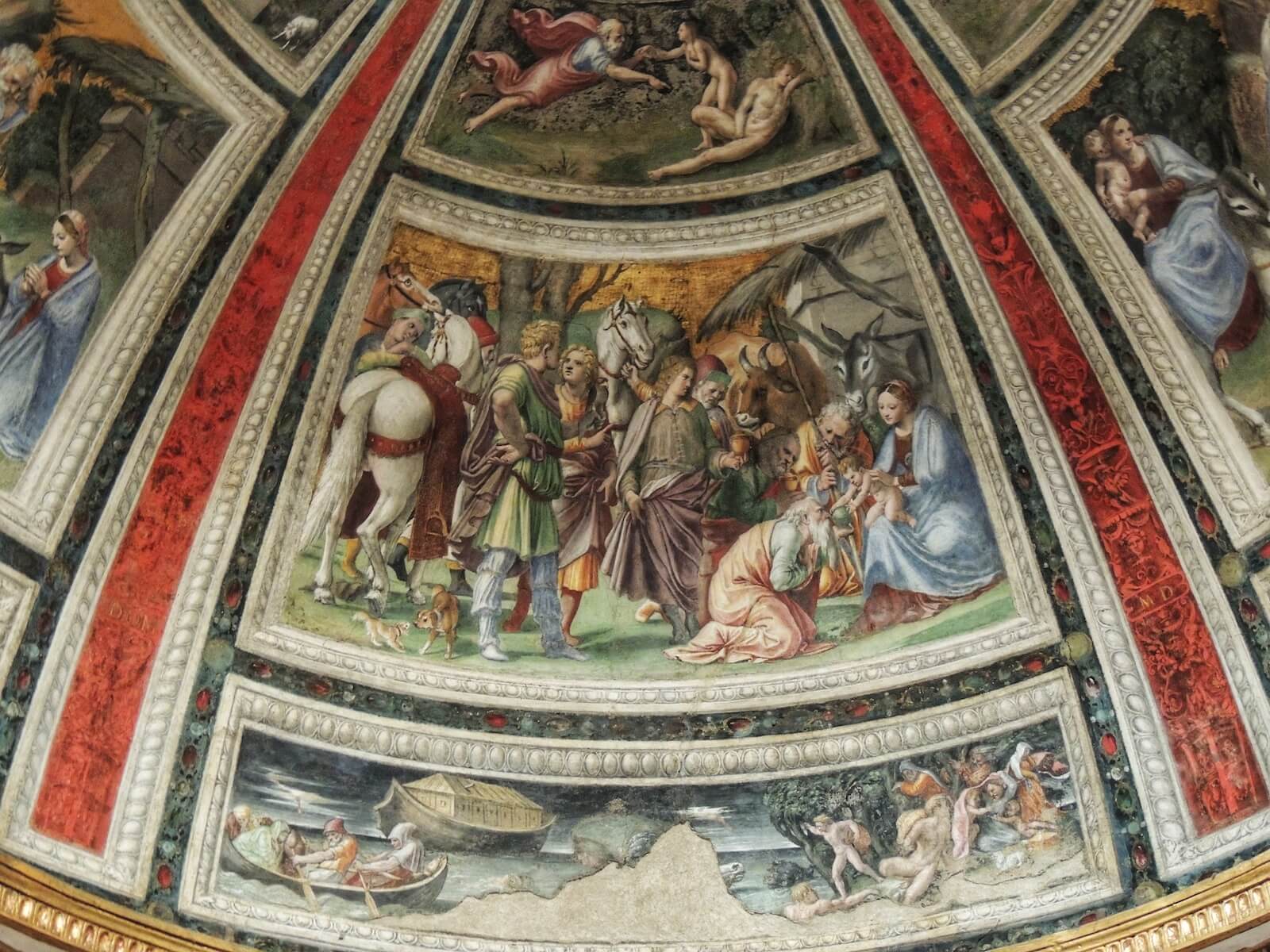This image captures the intricate and ornate ceiling of an architectural marvel, possibly a church or museum, with a distinct biblical theme. Dominating the scene is an opulent arched dome decorated with vibrant artwork meticulously framed in tan trim. The central piece of the ceiling showcases an elaborate tableau featuring a white horse facing backward and a group of people, including a kneeling woman before a figure that might be holding a baby, suggestive of Mary and Joseph. Surrounding this scene, some individuals wear long, flowing robes in shades of green, red, blue, and brown, adding to the rich color palette.

Flanking the central artwork are vertical red stripes, narrowing as they ascend, interspersed with swirls of color and sections of blue. Above and below the main picture are additional images, with the top section depicting more biblical characters, including what appears to be people floating in the air. The lower section has a depiction of people in a rowboat, set against what might be a partially destroyed scene or naturally sandy ground, adding a rustic, historical texture to the presentation. The entirety of the ceiling's artwork is enveloped by a combination of white and blue borders that frame each segment, presenting a vivid, almost Sistine Chapel-like visual narrative, rich in religious symbolism and historical context.